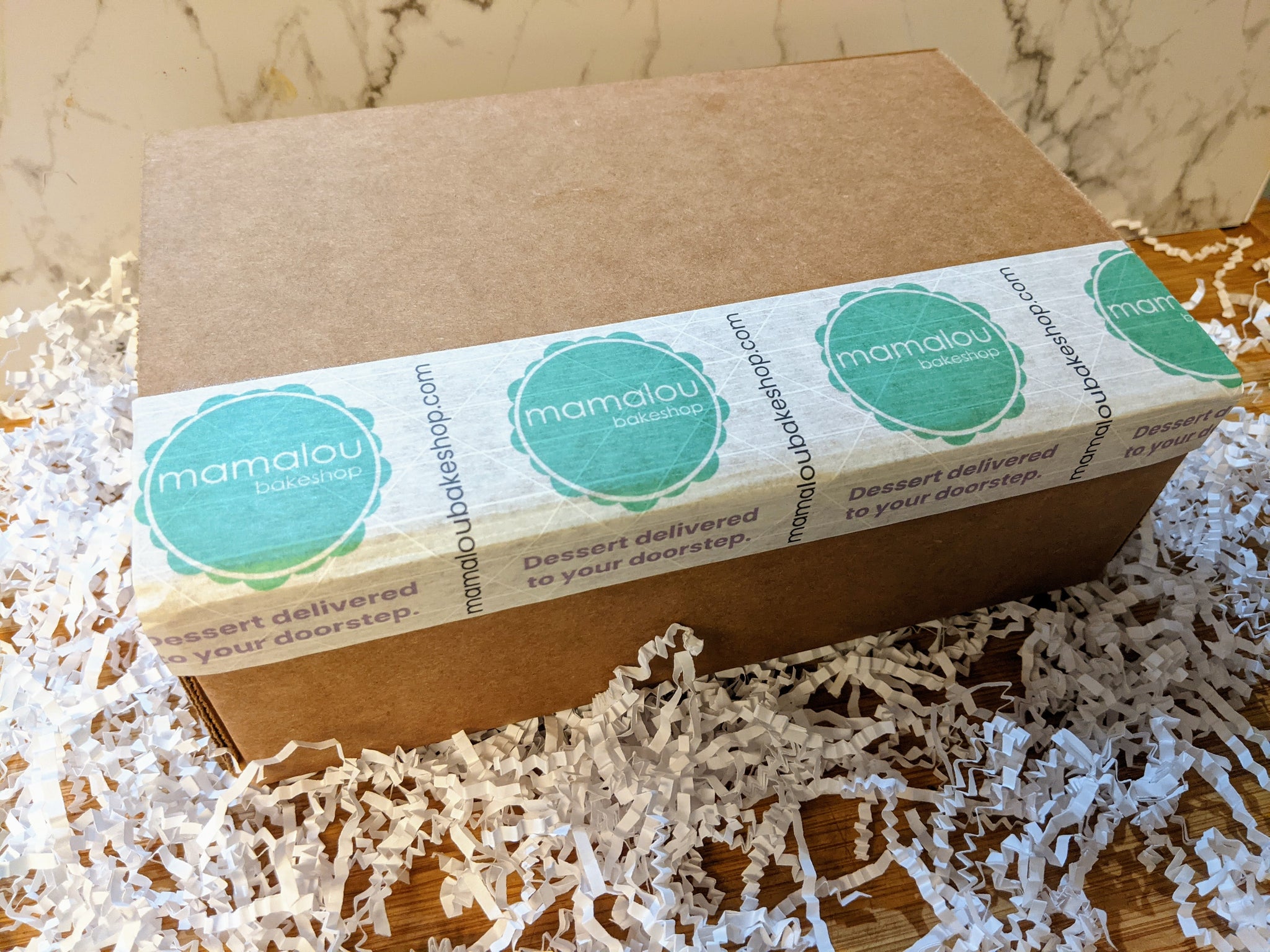A brown cardboard box, placed diagonally at the center of a wooden table, sits against a marble wall backdrop. The box is adorned with a distinctive white band featuring pale blue, medallion-style circles, each containing the name "Mama Lou" in white lettering. Below this, though somewhat illegible, is the subtitle "Bake Shop." The band acts as a sealing tape, continuing onto the front side of the box and displaying in gray lettering, "Dessert Delivered to Your Doorstep." The blue circles are consistently separated by lines of gray text, including the website "MamalooBakeshop.com," which appears both horizontally and vertically. Scattered around the base of the box is a layer of crimped white confetti paper, adding to the presentation's decorative touch. The overall setting suggests a thoughtful and elegant packaging for baked goods delivered straight to one's home.